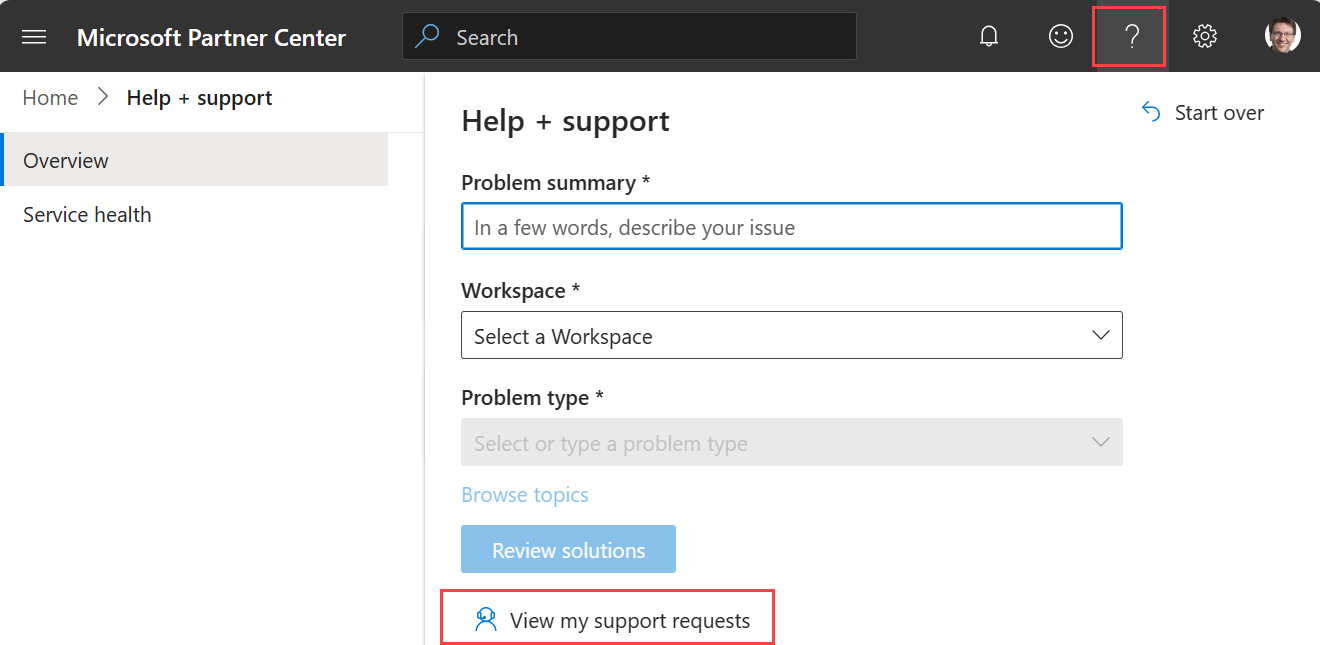The screenshot displays an interface from the Microsoft Partner Center. At the top, there is a black header on a white background. On the upper left side of the header, "Microsoft Partner Center" is written in bold white text. Adjacent to this, towards the middle, there is a black search bar with a blue magnifying glass icon. On the upper right corner of the header, several icons are visible: a notification bell, a smiley face, a question mark outlined in red, a settings button, and a user profile image. The user profile image features a woman with short brown hair and glasses.

Below the black header on the left side, there is gray text that reads "Home," followed by a right arrow, and "Help and Support." Beneath this is a gray box that contains the word "Overview," and below that, another link titled "Service Health."

Centered on the page, just below the black header, the words "Help and Support" are prominently displayed in bold black text. Directly underneath this heading is a form section. The first field in the form is labeled "Problem Summary" with an asterisk indicating a required field. The input box is outlined in blue and has placeholder text that instructs users to "In a few words, describe your issue."